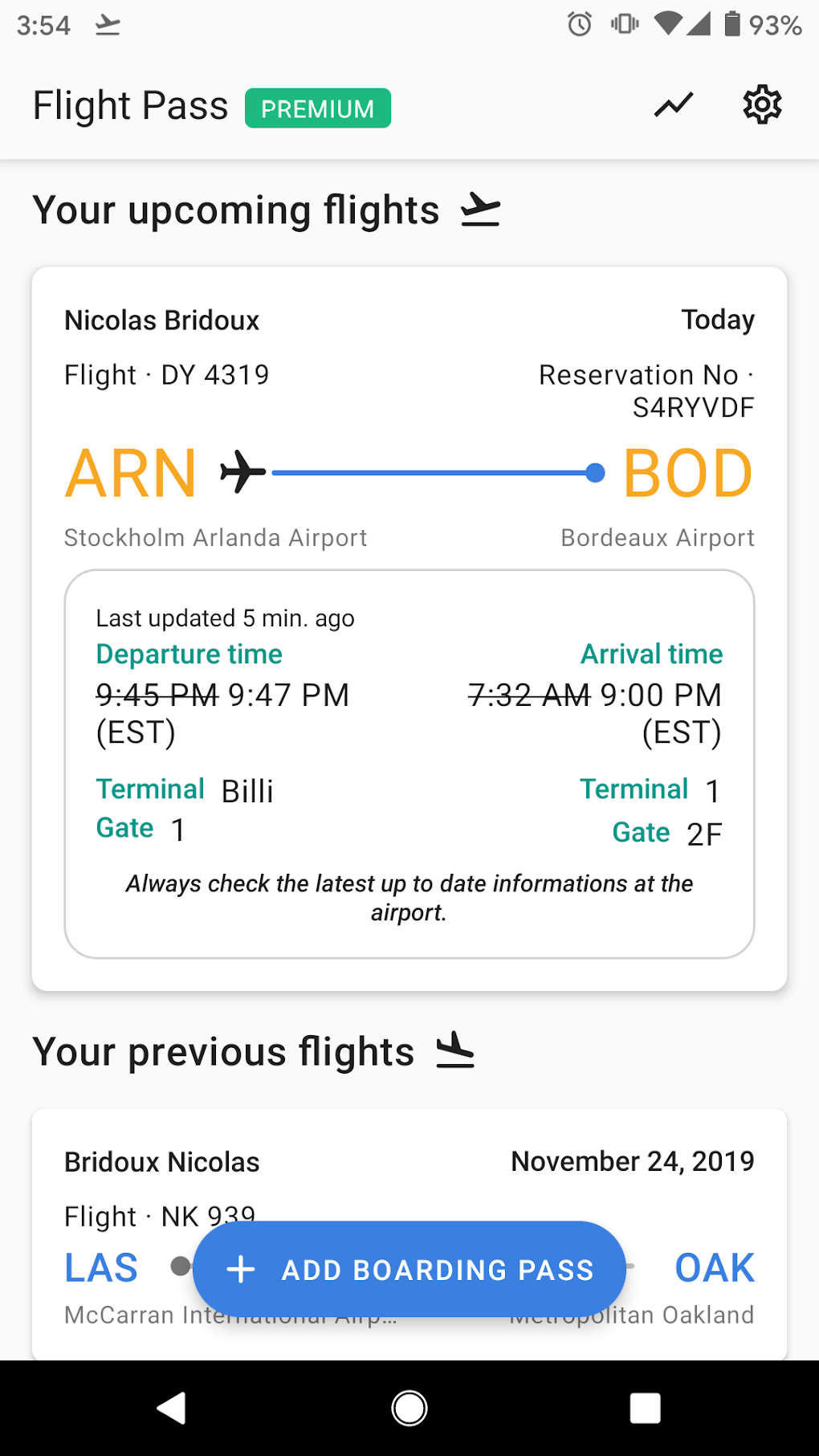This mobile phone screenshot details a flight pass. The interface displays the time at the top left corner, while the top right corner shows various icons and a battery level of 93%. The address bar reads "flight pass" with a green "premium" box adjacent to it.

The screen lists upcoming flights, highlighted by a plane icon, with a grey-outlined section containing passenger details. The passenger is Nicholas Bridoux (B-R-I-D-O-U-X), and the flight is scheduled for today. Flight number DY4319, linked to reservation number S4RYVDF, is shown. The departure airport code ARN (Stockholm Arlanda Airport) is on the left, followed by a plane icon and a blue line leading to the arrival airport code BOD (Bordeaux Airport).

Below this section, it indicates "last updated five minutes ago." The original departure time of 9:45 PM has been crossed off and updated to 9:47 PM. Similarly, the arrival time has been adjusted from 7:32 AM to 9:00 PM EST. Departure and arrival terminals are listed as Terminal 1, Gate 2F. 

A reminder to "always check the latest up-to-date information at the airport" is prominently displayed. At the bottom of the image, previous flights are listed, including a trip from LAS (Las Vegas) to OAK (Oakland). Above this section, there is a blue horizontal oval button with "Add boarding pass" in white text and a plus icon.

Finally, the bottom of the image features a black strip containing three icons, providing additional navigation options.